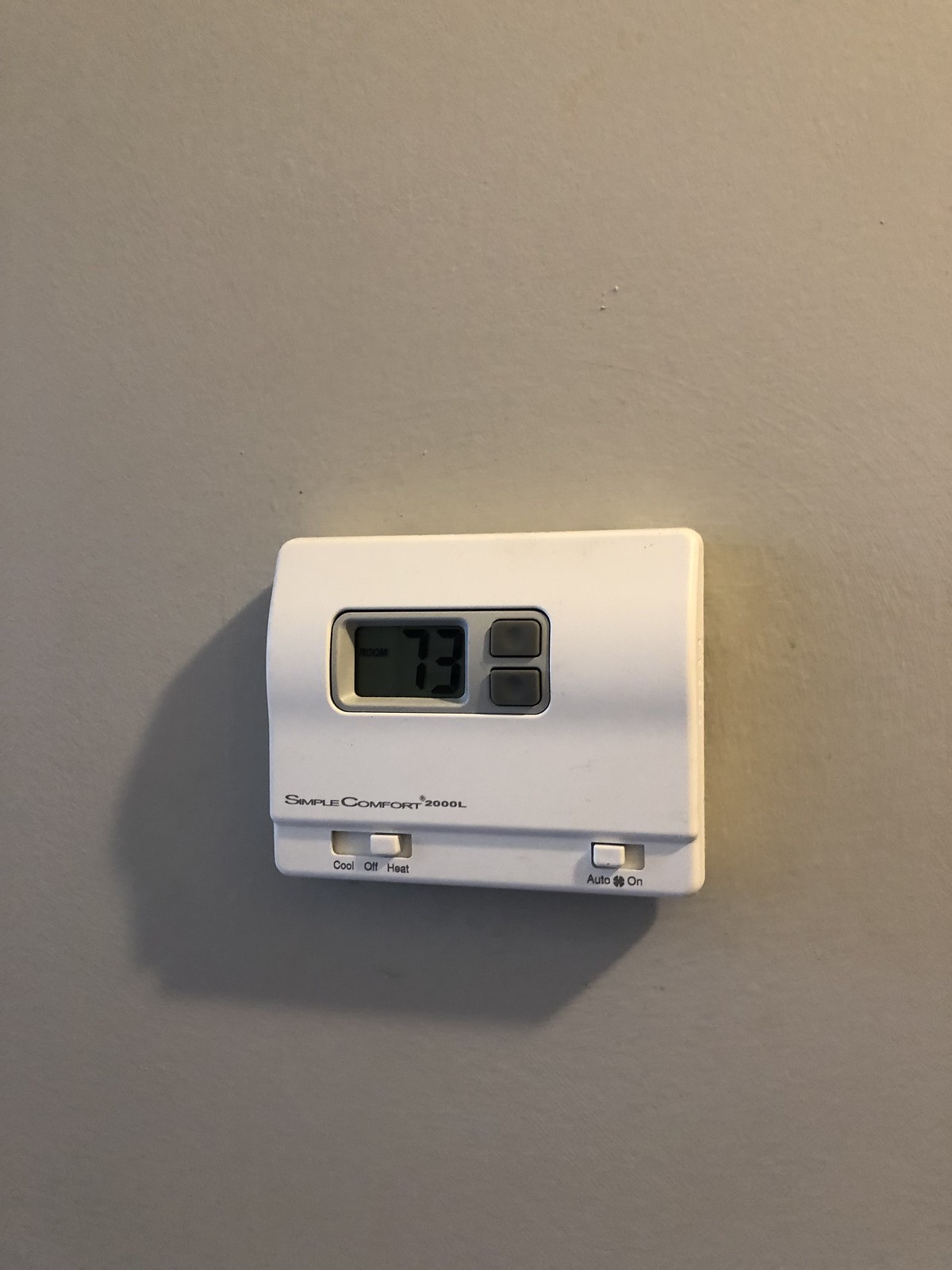The image depicts a thermostat affixed to a wall, which is painted in a uniform shade of ivory. The wall has a smooth yet slightly textured surface, and the entire scene is illuminated by artificial light, casting a shadow of the thermostat to the bottom left.

Positioned centrally and slightly below the midpoint of the image, the thermostat is made of a white plastic material and features a predominantly flat rectangular shape. Approximately one-third down from the top, the thermostat has a raised section, a small bump that extends outward before flattening again. Embedded within this raised area is a gray rectangle with rounded edges. This inset contains a small, dark gray screen displaying the word "ROOM" in capital letters, followed by the number "73" in black font.

Below the screen, two protruding buttons allow for temperature adjustments, marked for increasing and decreasing the temperature. At the bottom of the thermostat, the text "Sample Comfort 2000 L" is inscribed. Additionally, there are two white switches below this text, used to toggle between settings: "Cool," "Off," "Heat," and "Auto," "On."